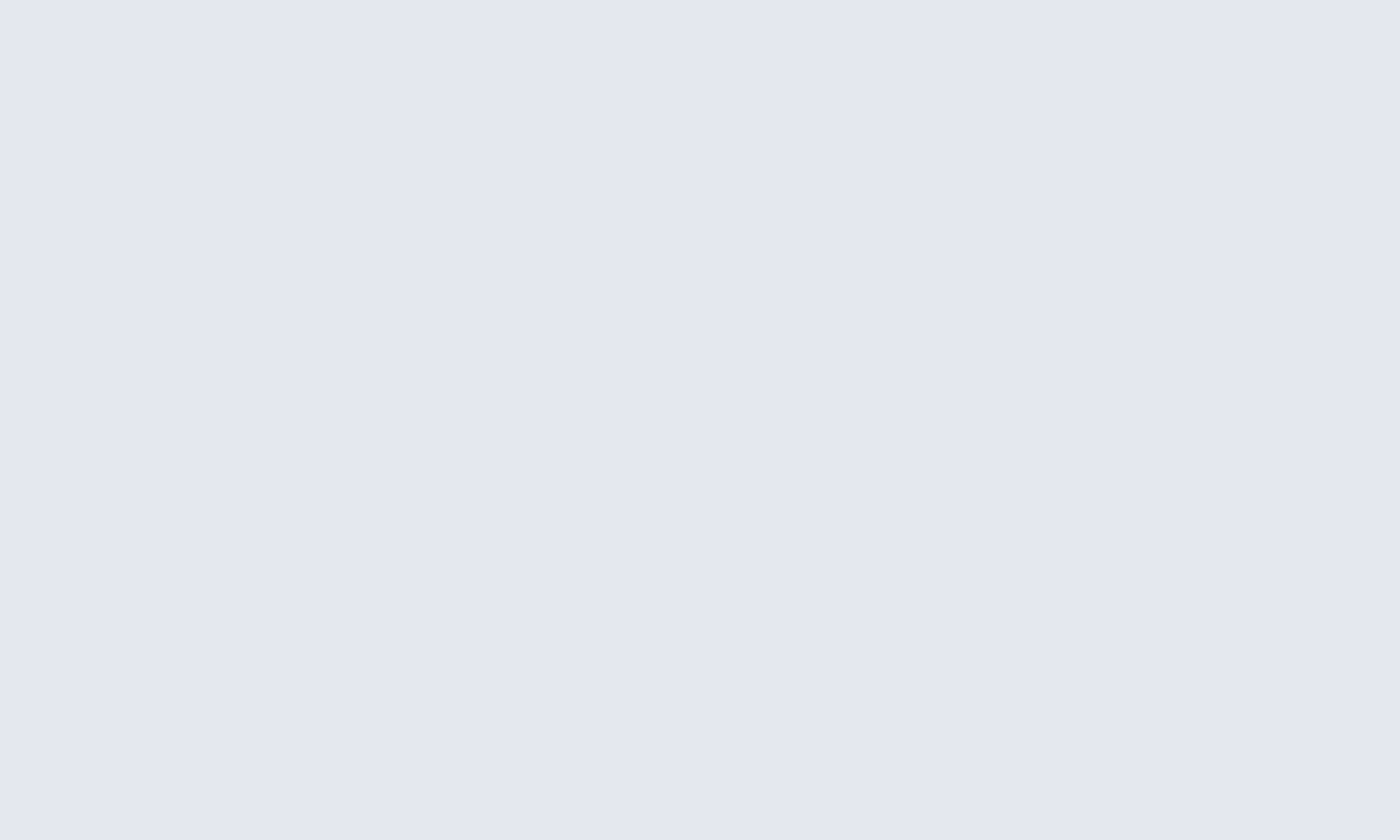This image presents a blank canvas, marked only by a plain, light gray square. There are no distinguishable objects, text, or numerical elements within the confines of this rectangular frame. Its neutral tone suggests an off-white or very light gray color, devoid of any additional features that could provide context or deeper meaning. The simplicity and emptiness may evoke a sense of minimalism or absolute abstraction. There is no background, no subtle details, and no discernible elements to analyze. This image serves as an unembellished expanse, offering a sense of stillness and silence. It almost functions as a placeholder, devoid of content yet full of potential, inviting the curiosity and imagination of the viewer to project their own interpretations or await further input.